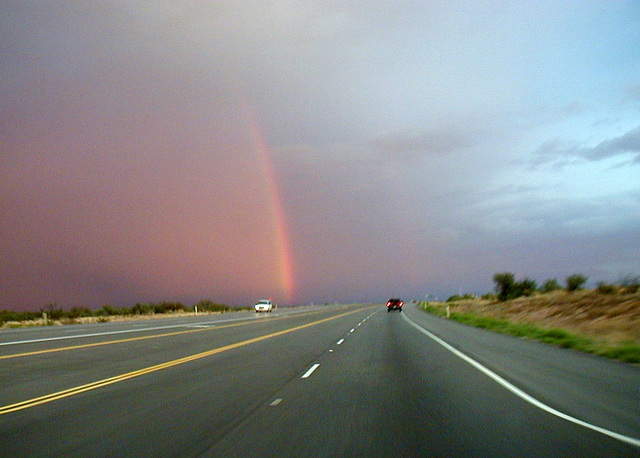The photograph captures the view from a car driving down a four-lane highway with a central yellow dividing lane. The road appears freshly wet, perhaps following a recent rain, reflecting the overcast sky. Up ahead, a dark-colored truck is seen traveling farther down the same direction, its taillights aglow. On the opposite side of the road, a white truck moves toward the camera. Flanking both sides of the highway is low vegetation, mainly brown and green bushes, with no tall trees in sight.

The sky is a striking feature in this image. It is split into two tones: the right side is a conventional light blue with scattered clouds, while the left side is painted with hues of pink and yellow, suggesting a recent sunset or the influence of the rainbow. Dominating this section is a vivid rainbow arching upward from the horizon toward the top of the frame, displaying distinct red, yellow, and green stripes. The rainbow's presence adds a surreal quality to the scene, contrasting beautifully against the darker, pinkish sky on the left.